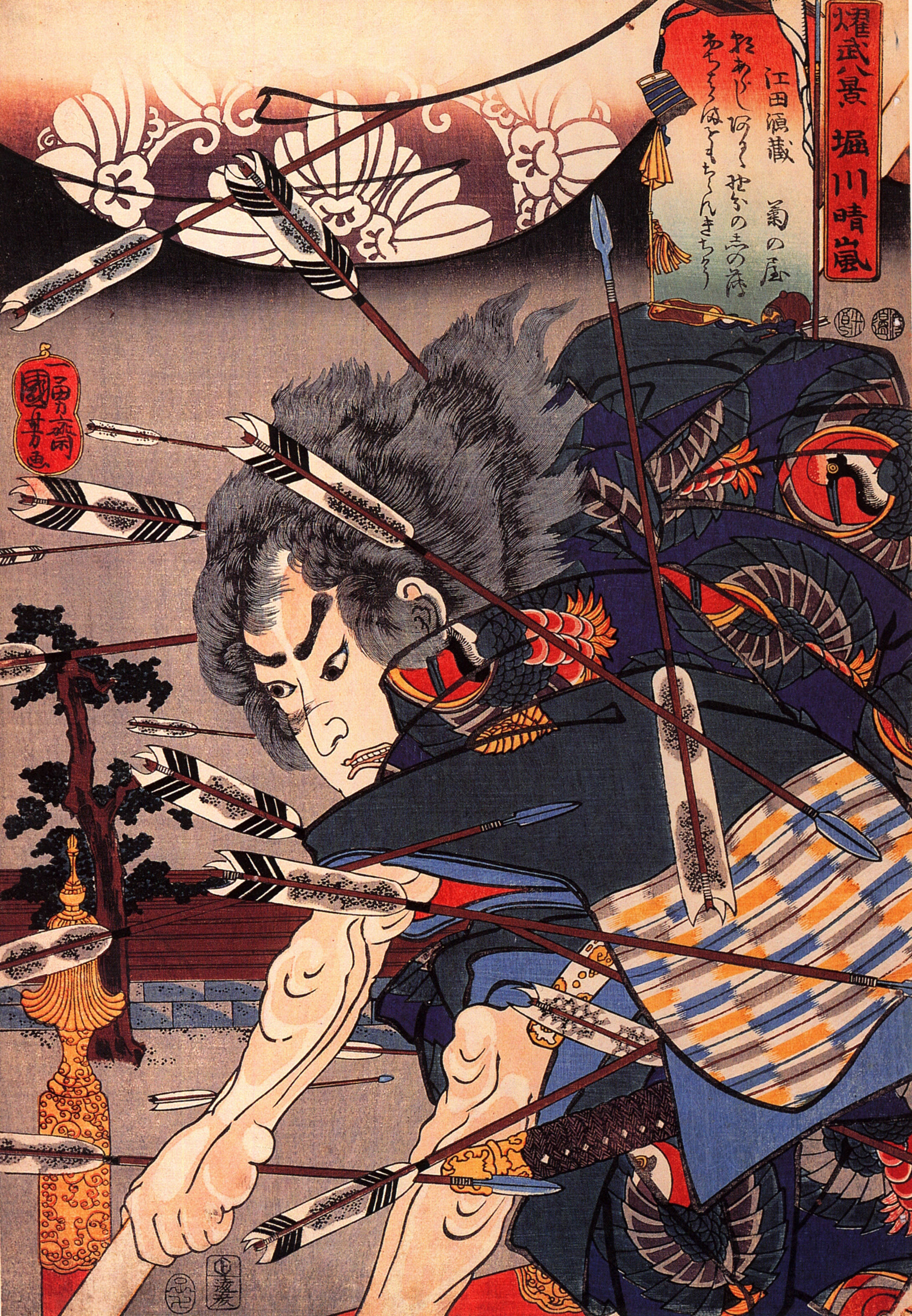This vibrant and intricate painting depicts a Japanese samurai warrior captured in a dramatic and action-filled moment. The central figure, rendered in bold black lines, exhibits classic Japanese facial features with angry, slanting eyebrows. His long, fluffy hair flows backwards in layers, painted in shades of gray and black, heightening the sense of movement.

The samurai is positioned front and center, slightly crouched with one knee visible and his arms outstretched, possibly holding an unseen weapon. He wears a luxurious navy blue kimono adorned with ornate red, gold, and gray designs, including patterns of birds woven into the fabric. The sleeves of this elaborate garment are light blue, complemented by gold details.

Around the warrior, arrows are seen in mid-flight, some appearing to hit their mark, adding to the dynamic tension of the scene. The background is a muted gray, allowing the detailed figure to stand out vividly. The painting is taller than it is wide, emphasizing the vertical composition. In the top right corner, Asian text, likely Japanese, descends vertically, accompanied by traditional designs, adding to the authenticity and richness of the artwork.